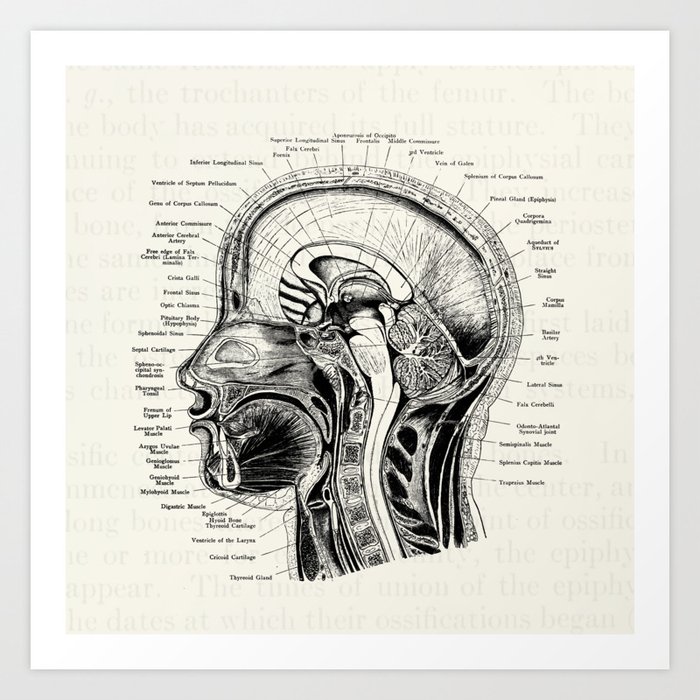This image appears to be a detailed diagram from a textbook, depicting the left side view of a human head in an almost x-ray form against a light grayish background. The diagram is rendered in grayscale, featuring intricate sketches of the skull, muscles, and organs. Surrounding the head are numerous labels, over 25 to 30, each connected by arrows pointing to specific parts within the head, such as the thyroid gland. The labels, however, are quite small and challenging to read. The background contains faint, barely visible text, and the entire image is framed by a white border, which is further enclosed by an additional light gray square border.